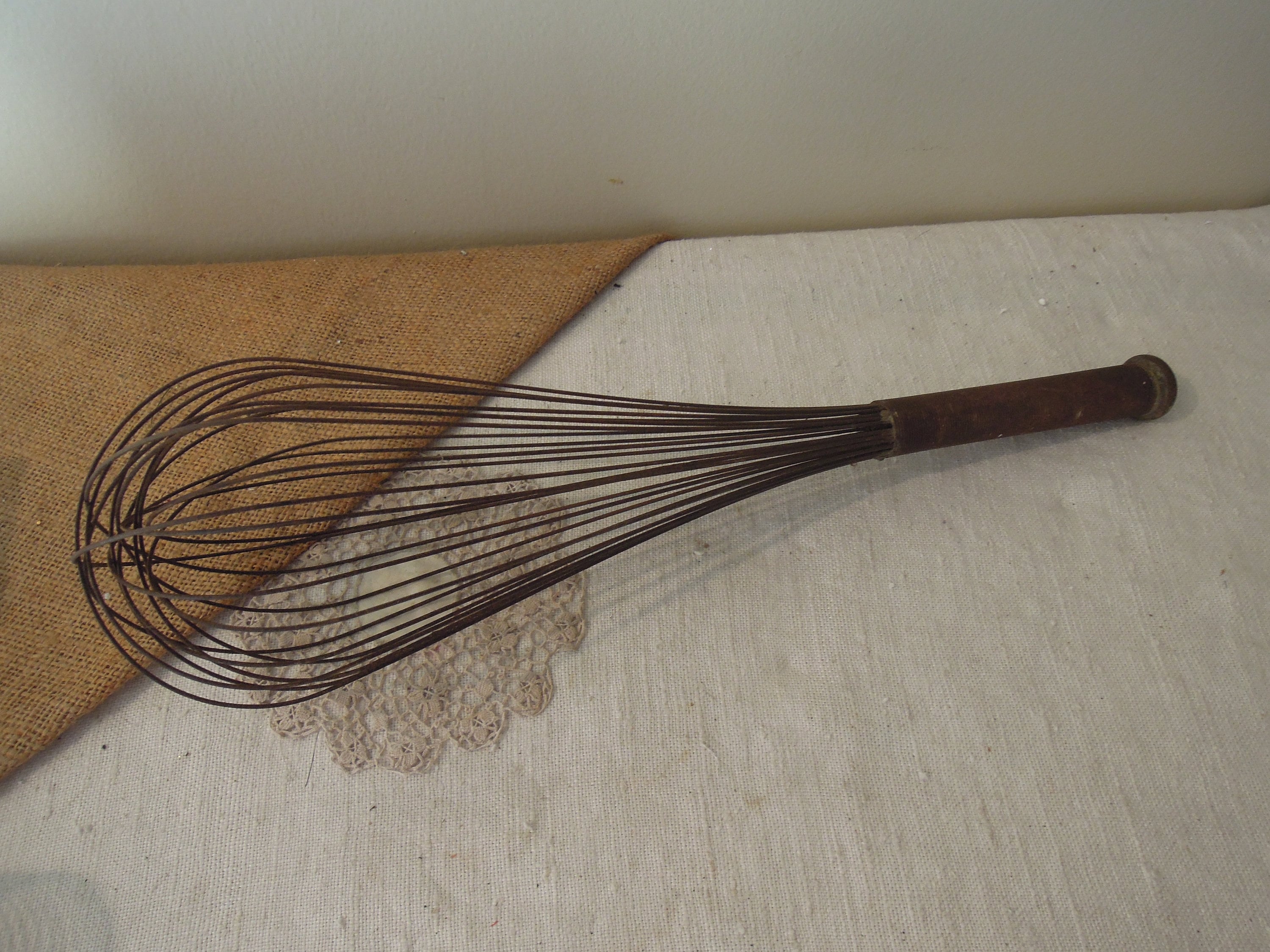The image depicts a rustic kitchen scene with an aged, rusty brown metal whisk resting on its side on a table. The table is covered mostly with a white, possibly linen tablecloth, but a brown, burlap fabric piece also runs diagonally across the left corner. A cream-colored, intricately embroidered flower doily lies partially beneath the burlap, with its white center visible against the white tablecloth. The whisk, with its many overlapping wires forming the stirring part, is positioned such that it spans across the cream-colored fabric and might extend onto the burlap. The setting is indoors, with the background featuring a simple white wall.